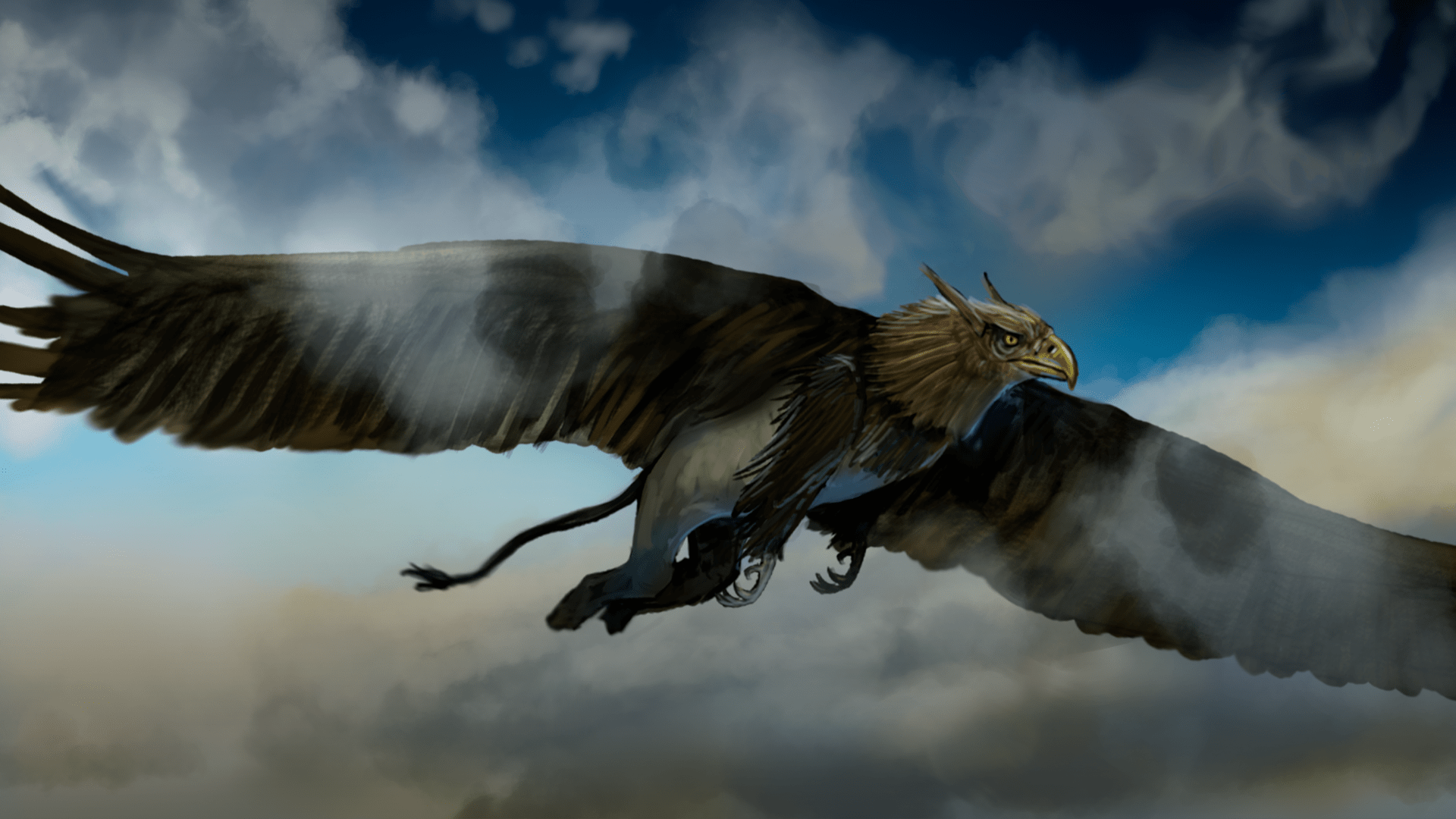This horizontal digital artwork portrays a massive eagle-like creature soaring in the sky. The focus is on this extraordinary beast with its enormous wings outstretched, spanning the entire width of the image from one edge to the other. The eagle's head, featuring a light gold beak and a single fierce yellow eye, is turned to the right in profile, showcasing its intense gaze and pointy ears tucked back behind its head. This creature is embellished with unusual attributes: its front legs end in large claws, while its back legs resemble hooves, and it has a long tail that bifurcates at the end, adding to its mythical appearance.

The sky behind the creature is rich with detail, transitioning from deep blues at the top to lighter blue streaks and an expansive cloud cover below. Wispy clouds add texture to the upper part of the background. The clouds themselves are predominantly white with hints of gray, giving a foggy impression. This scene combines the majestic and the mystical in a captivating aerial dance.